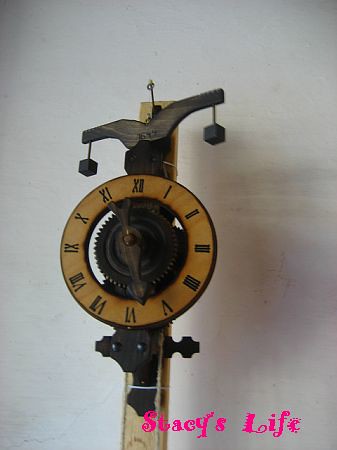This photograph features an intricately designed clock mounted on a wooden post against a white wall. In the bottom right corner, the phrase "Stacy's Life" is written in playful pink text, adding a personal touch to the image. The clock itself is a fascinating wooden circular disc with its interior cut out, revealing the mechanical workings inside. The clock hands are elaborately redesigned, showcasing fine craftsmanship.

The clock is attached to a darker wooden post, which is further supported by another darker wooden post, creating a sturdy structure. There are two black cube structures hanging from the top of the main wooden post, one on each side, adding to the clock's complex design.

The clock face features Roman numerals to indicate the time, enhancing its classical appearance. Below the clock, the year "1644" is inscribed on the post, possibly hinting at the clock's historical significance. The combination of unique elements and detailed design makes this photograph a compelling portrayal of both artistry and history.